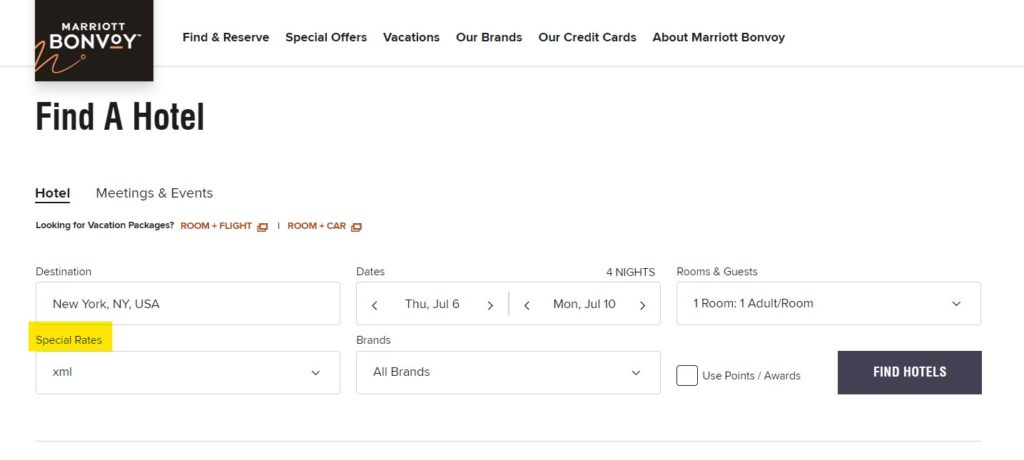The image showcases the Marriott Bonvoy logo, displayed prominently in white text on a horizontally extended black rectangle. "Bonvoy" appears as the largest font on this rectangle. To the right of the logo, the following options are listed in a clean, organized manner: "Find and Reserve," "Special Offers," "Vacations," "Our Brands," "Our Credit Cards," and "About Marriott Bonvoy." Below this is a fine gray line, serving as a neat separator.

On the left side, the largest text reads "Find a Hotel" in bold black font. Adjacent to this, two tabs are visible: "Hotels" and "Meetings and Events." The "Hotels" tab is underlined and displayed in black, indicating the current selection, while the "Meetings and Events" tab is in gray.

Underneath these tabs, there's a prompt reading "Looking for Vacation Rental?" followed by two clickable links, "Room + Flight" and "Room + Car," highlighted in brown. Further down, a labeled data field for "Destination" is filled with "New York, New York, USA."

A yellow button labeled "Special Rates" is situated below this entry field. Beside this, there is an option for "XML," which includes a drop-down menu.

To the right, details for "Dates" are specified: the field indicates a "Four Nights" stay, with the actual dates listed as "Thursday, July 6th through Monday, July 10th." Finally, there is an option labeled "Brands," set to "All Brands," accompanied by another drop-down menu for selection.